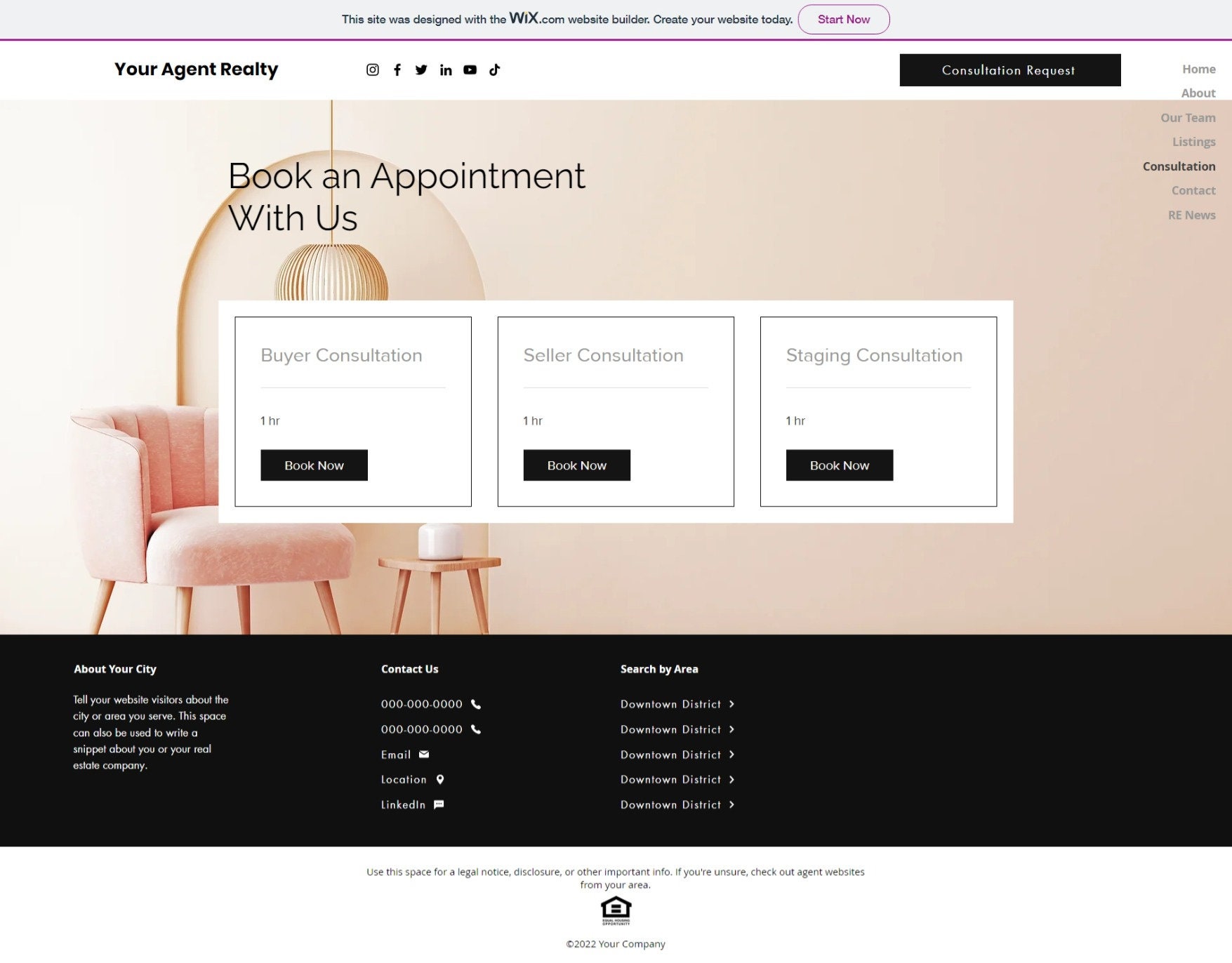**Descriptive Caption:**

The webpage for a realty agent is thoughtfully designed to facilitate booking appointments. The layout is primarily landscape and rectangular, incorporating several distinct layers to guide the user. 

The background is a slightly lighter pinkish-salmon color, suggesting a cozy living room setting. Within this living room, located on the left side, there's a pink chair with wooden legs, an end table also with wooden legs, and a hanging lamp above the chair.

Central to the page is an important white rectangular section divided into three squares. Each square presents a different service: 
- The left square: "Buyer Consultation"
- The center square: "Seller Consultation"
- The right square: "Staging Consultation"

Beneath each square, there's a black rectangle with the white text "Book Now."

The bottom section of the image, occupying roughly the last 20-25% of the page, features a long black rectangle with left-justified white text. This section is divided into three parts:
- The left portion titled "About Your City" with a five-line descriptive paragraph below.
- The middle portion titled "Contact Us" featuring placeholder information like phone numbers (000-000-0000), an email, and LinkedIn link.
- The right portion titled "Search By Area" listing five clickable areas like "Downtown District" with arrows.

At the very top, there's a thin light gray rectangle with the text "This site was designed with a wix.com website builder – create your own website today," and a clickable button labeled "Start Now." Below that is a purplish-red line extending across the whole width of the page.

In the upper left corner within a white section, "Your Agent Realty" is written in black text. Adjacent to it are social media icons for Facebook and Twitter. To the far right, a black box with the white text "Consultation Requests" serves as another clickable feature to schedule consultations.

Overall, the webpage is well-structured to assist visitors in booking various types of consultations with ease while providing essential contact and locale information.